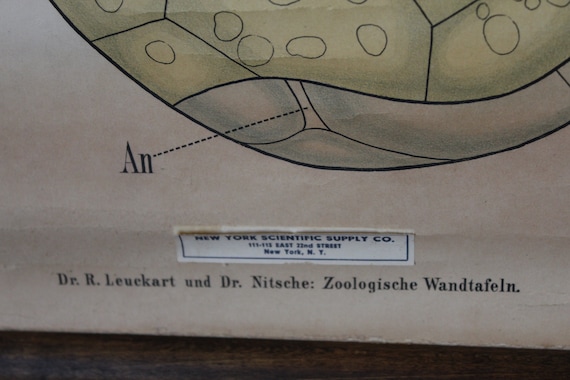The image depicts a zoological diagram, attributed to Dr. R. Leuckart and Dr. Nischke, with professional affiliations that appear in non-English text beneath their names. The diagram is set against a light brown background and is partially resting on a light brown table, slightly visible at the bottom of the image. Central to the diagram is a rounded, possibly cell-like or turtle-shaped structure, segmented with demarcating lines and colored in shades of green and blue. Key features within this structure include squares and circles, with one section labeled 'AN' pointing to the center. The top right of the diagram features this round structure prominently, while a white box at the center gives credit to the New York Scientific Supply Company. Overall, the diagram appears complex and specialized, likely pertaining to the field of zoology.